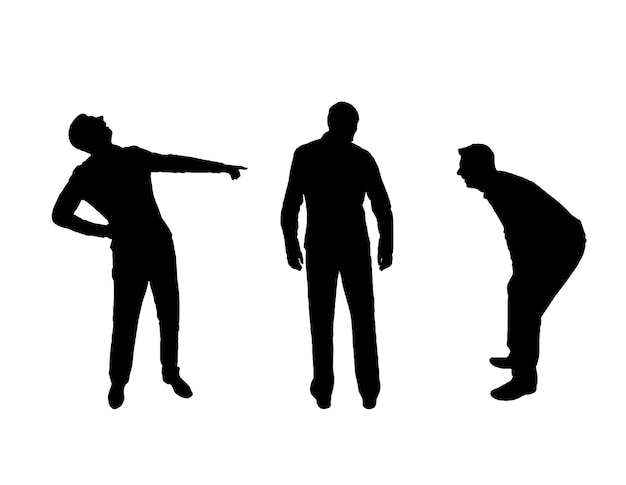In this image set against a stark white background, three men are depicted entirely in black silhouettes, obscuring any facial features or clothing details. The man on the left, standing with his right arm on his hip and his head thrown back as if laughing, points his left arm towards the man in the center. The central figure stands with his arms hanging straight down by his sides, his back to the viewer, and his head slightly turned to the right. On the right, the third man is shown from a side profile, facing the center. He is bent over, with his hands placed on his knees, giving the impression that he too is laughing or smiling at the man in the center. The composition creates a dynamic interaction, focusing on the reactions of the men on the left and right towards the central figure.